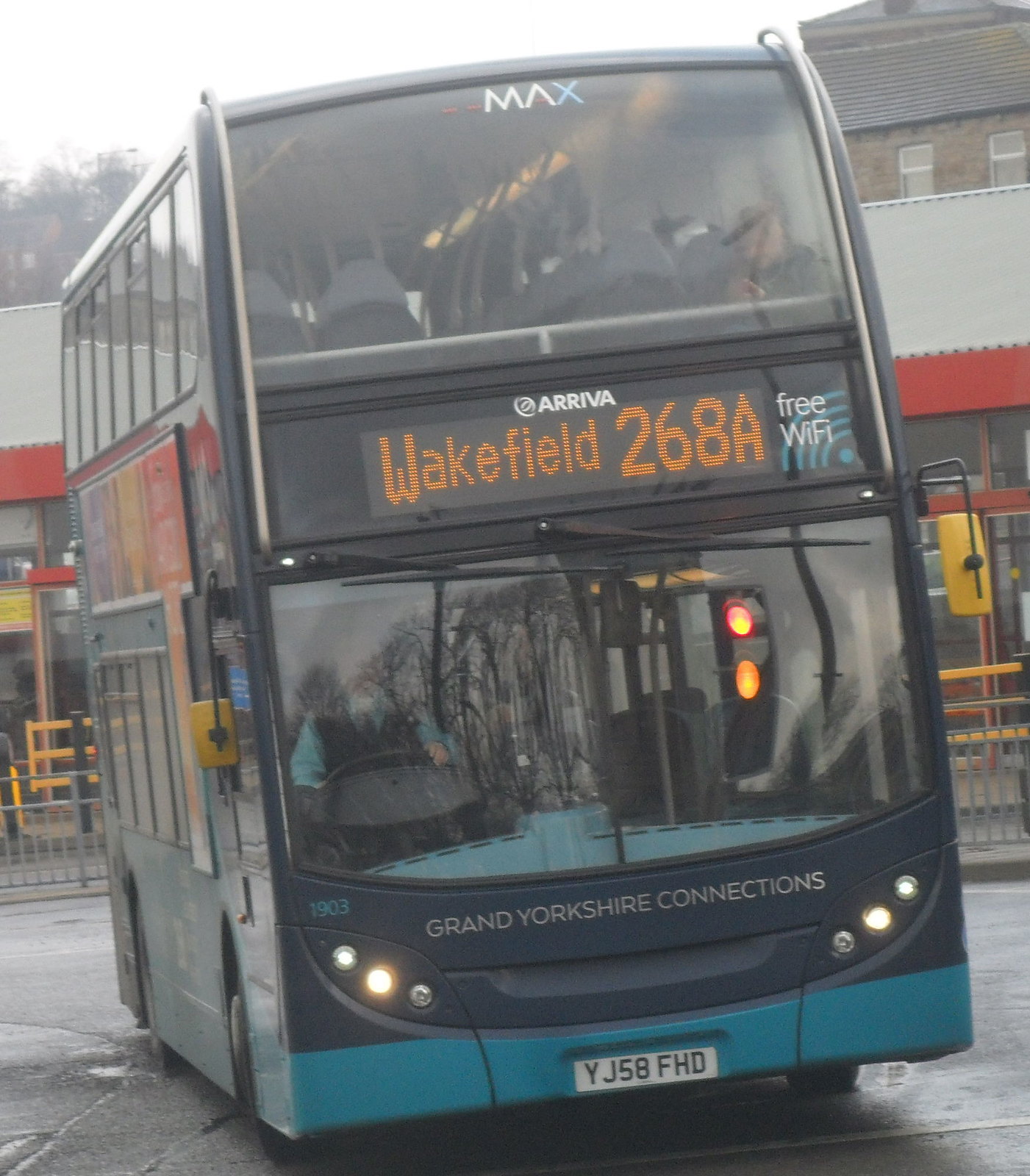This outdoor photograph showcases a dynamic scene of a large double-decker bus in motion. The bus, prominently colored in dark blue with turquoise accents, features numerous windows across both its main and upper levels, indicative of its double-decker structure. The frontal view highlights a digital destination readout displaying "Wakefield 268A" and "free Wi-Fi," along with the bussing company's name, Arriva, near the top, separating the windows of the two levels. The bus's lower front section bears the branding "Grand Yorkshire Connections," and below this, the headlights are illuminated, casting a soft glow, with the license plate reading YJ58 FHD.

From the image, details such as three frontal lights and yellow side mirrors are noticeable. The driver, visible through the large frontal windows, is wearing a tie and turquoise shirt, while a couple of passengers can be seen seated on the upper level. There is also a reflected scene in the main-level window suggesting a gray and red building background, consistent with a row of stores.

The roadway beneath appears wet, suggesting recent rain or morning dew, contributing to the reflections, including that of a traffic signal. Overall, the backdrop blends in with the urban environment, enhancing the dynamic and bustling atmosphere depicted in the photograph.